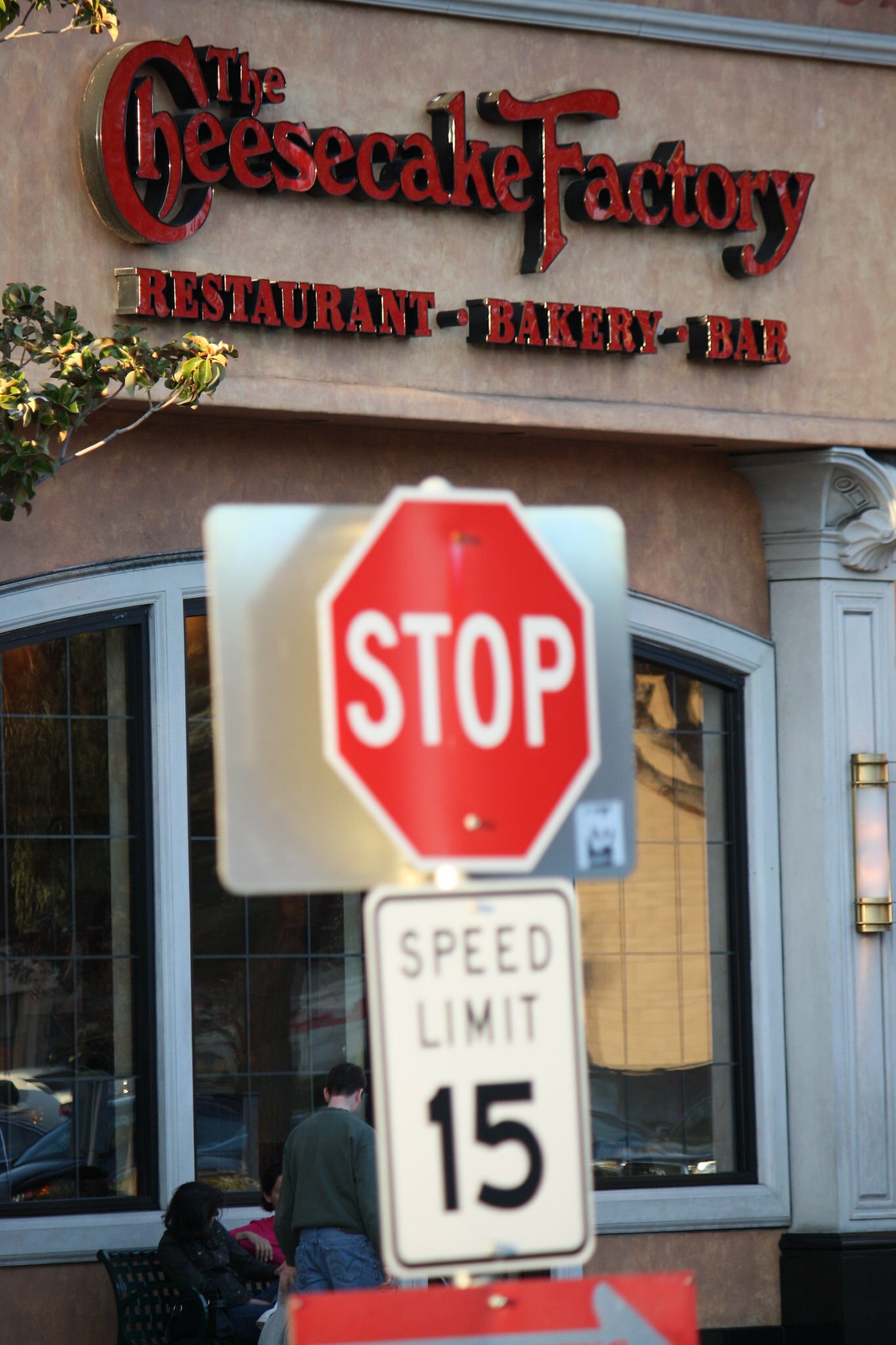In this detailed image captured outdoors during the daytime, the scene centers on the front of a Cheesecake Factory restaurant. The focus is dominated by a large red Cheesecake Factory sign with intricate lettering spelling out "Cheesecake Factory" across the top of the building. Underneath the main sign, additional text in red announces "Restaurant, Bakery, Bar." The façade of the building features large arched windows with grid patterns, resting against a textured brown stonework. 

In the immediate foreground, a stop sign is prominently positioned, nearly cutting through the center of the image. Directly beneath the red, octagonal stop sign is a white speed limit sign indicating a speed limit of 15. To the left of the signs, a silver backing suggests the presence of another sign, though its details are obscured. Toward the bottom left of the frame, a bench is visible with a couple of people seated, and a man walking past them. 

The color palette of the image includes a mix of tan, green, red, silver, gold, maroon, white, black, and gray, adding to the vibrancy and clarity of the photograph. The setting appears to be an outdoor area, likely just outside the restaurant, captured in the middle of the day. 

Overall, the composition smoothly juxtaposes the bustling street elements with the classic architecture and branding of the Cheesecake Factory, encapsulating a moment in an urban environment.